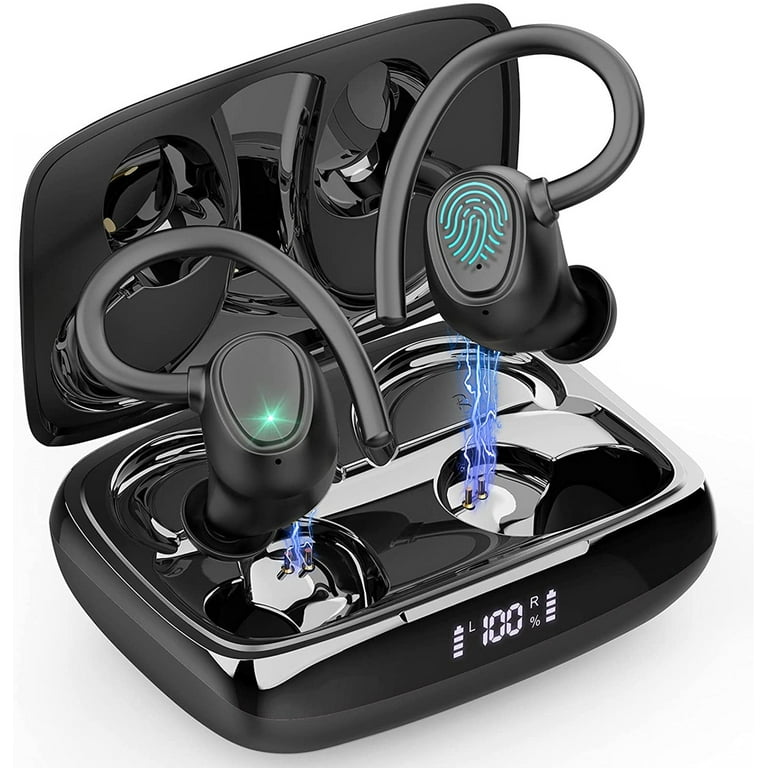The image depicts a sleek, modern, and innovative black earbud case with silver accents. The case features a digitized display on the front, which includes an L for the left earbud, an R for the right earbud, and a percentage sign indicating battery levels; a clear number 100 is shown between L and R, signifying full charge. The left side of the case has an icon signifying that the left earbud is fully charged, while the right side has a similar icon for the right earbud. Green markings and electrical lines from the case to the earbuds suggest the charging process. Inside the case, the earbuds are elevated for a better view. The left earbud is entirely black with a swirling design, while the right earbud features an emblazoned thumbprint design and also has a black swirl. These wireless Bluetooth in-ear headphones include hooks that go over the ears, eliminating the need for cords.